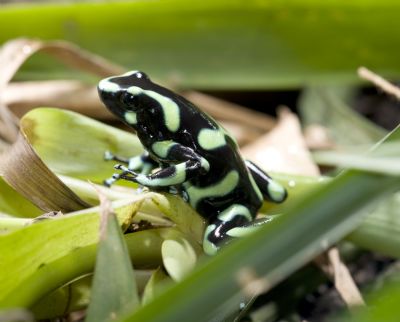The photograph captures a glossy and shiny poison dart frog, predominantly black with irregular neon green spots and faint light pastel green stripes. The frog is positioned in profile, facing upward to the left of the frame. It is perched on a mix of green foliage and brown, possibly dead, leaves, giving the scene a humid, damp, rainforest-like atmosphere. Both the frog's front feet and hind legs are visible, and its dark black eyes stand out prominently. The frog is in sharp focus, while the surrounding environment is softly blurred. The well-lit, landscape-mode image presents a detailed and vibrant view of this intriguing amphibian amidst its natural habitat.